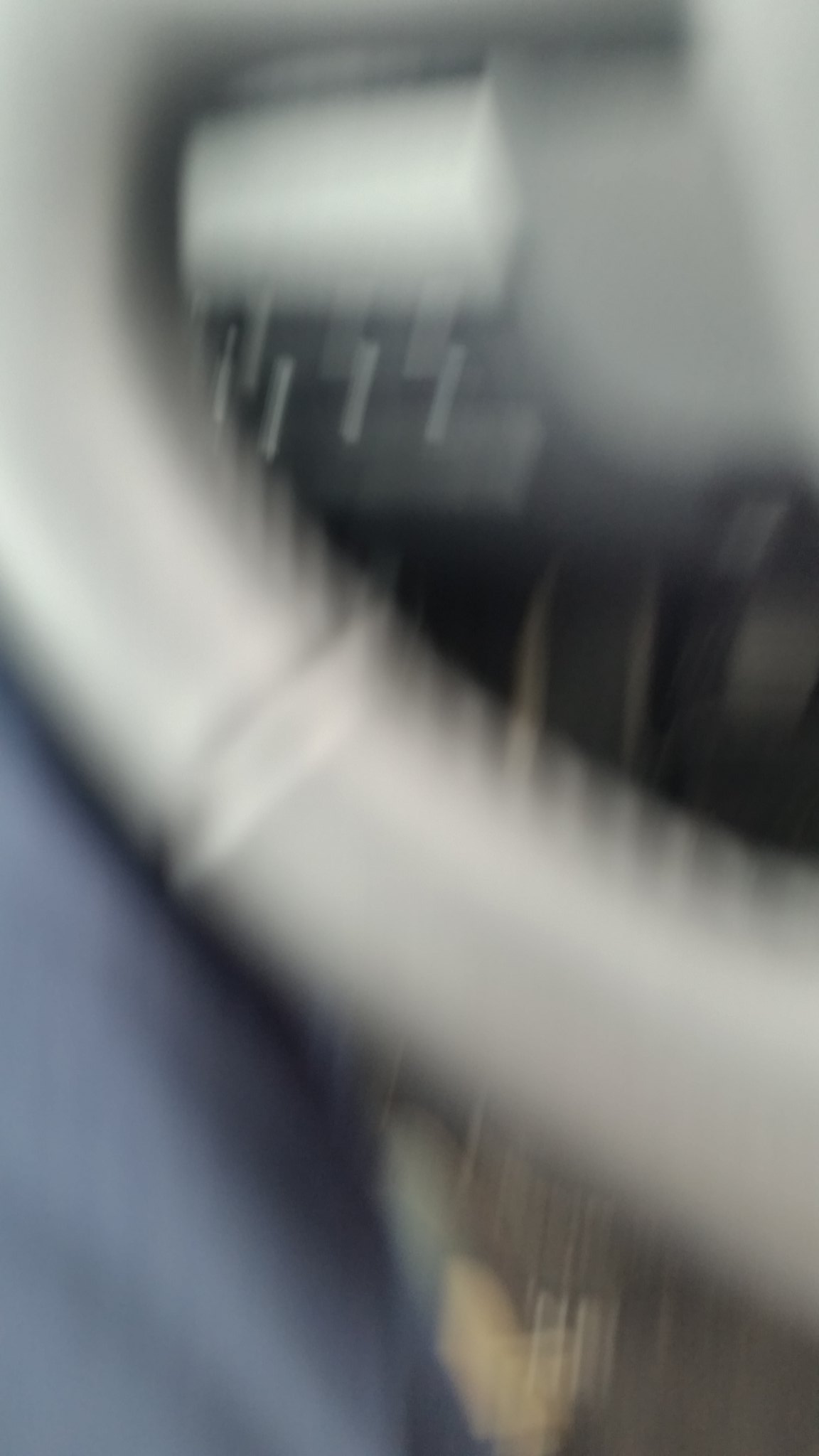This image captures an extremely blurry, close-up view inside a car, prominently featuring a gray steering wheel. The photograph focuses on the bottom left portion of the steering wheel, showing about 25% of its surface. Through the central gap of the wheel, a gas pedal is vaguely visible. In the lower left corner, there is a leg clad in blue jeans resting near the wheel. The floorboard beneath the wheel appears dark gray. Partial glimpses of the car’s dashboard and what seems to be a footrest are also apparent in the blur. The overall impression is of a hasty or accidentally taken photograph, resulting in a lack of clarity and detail.